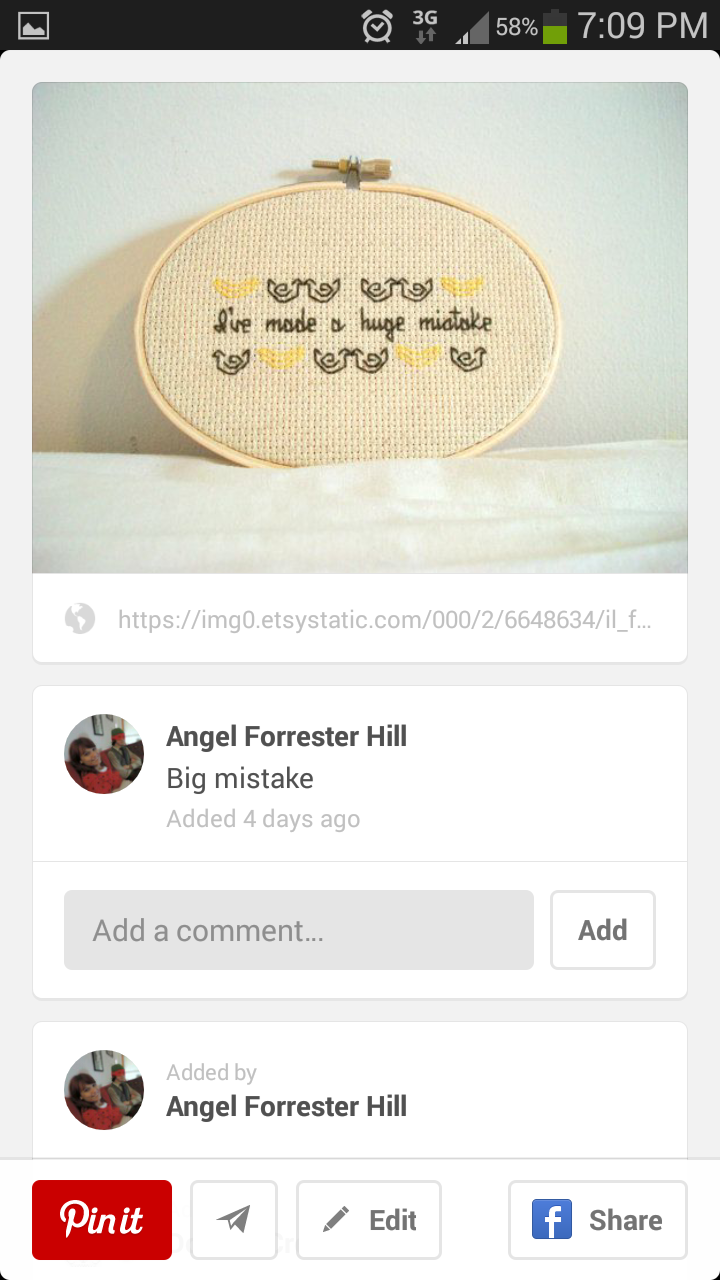The image appears to be a screenshot taken from an older Android smartphone, as indicated by the black header at the top showing icons such as an alarm, 3G with a couple of bars, and a 58% battery life at 7:09 p.m. This vertically oriented screenshot from Pinterest depicts an embroidery hoop with alternating yellow colors and the text "I've made a huge mistake" alongside an illustration of two little birds kissing. At the bottom, there's a URL indicating that this might be an Etsy image, reading, "https://img0.etsystatic.com/000/2/6648634/ilf." 

Beneath the embroidery photo, the post contains user interaction elements including a profile picture of two people sitting on a couch, identified as Angel Forrester Hill, who commented "big mistake" four days ago. More user interface elements include a red "Pin It" button, a paper airplane icon, an edit button represented by a pencil, and a Facebook share button. 

Below the primary comment by Angel Forrester Hill, there is another truncated comment indicating it is part of an ongoing conversation. Overall, the image encapsulates the social and interactive nature of Pinterest while also hinting at its origin from Etsy's website.